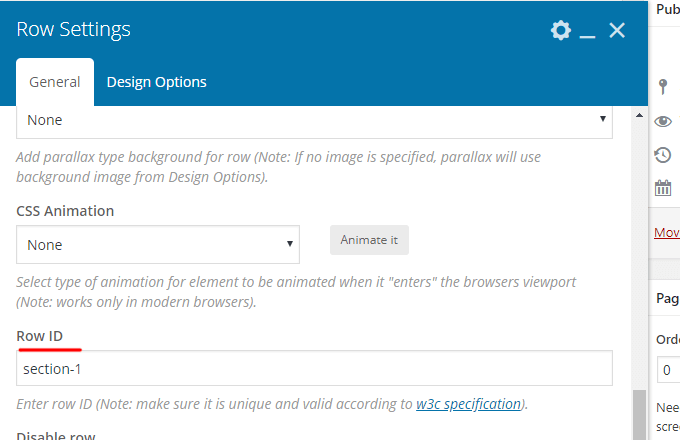This image displays a web page interface with a distinct blue border along the top. In the upper left corner, white text reads "Row Settings." On the upper right corner, there are two icons: a gear for accessing settings and an 'X' for closing the page. Below this blue border, a white tab area is visible with the word "General" highlighted, along with an adjacent option labeled "Design Options."

The main content of the page includes instructions and options for customizing a webpage row. The first instruction is to "Add parallax type background for row," noting that if no image is specified, the background from the design options will be used. Further down, it includes a section for "CSS Animation" that is currently set to "None," with a button labeled "Animate It" for adding animations. It explains that the selected animations will trigger when the element enters the browser's viewport, functioning only in modern browsers. Additionally, there is a "Row ID" field set to "section-1," with a note that users should enter a unique and valid row ID according to W3C specifications.